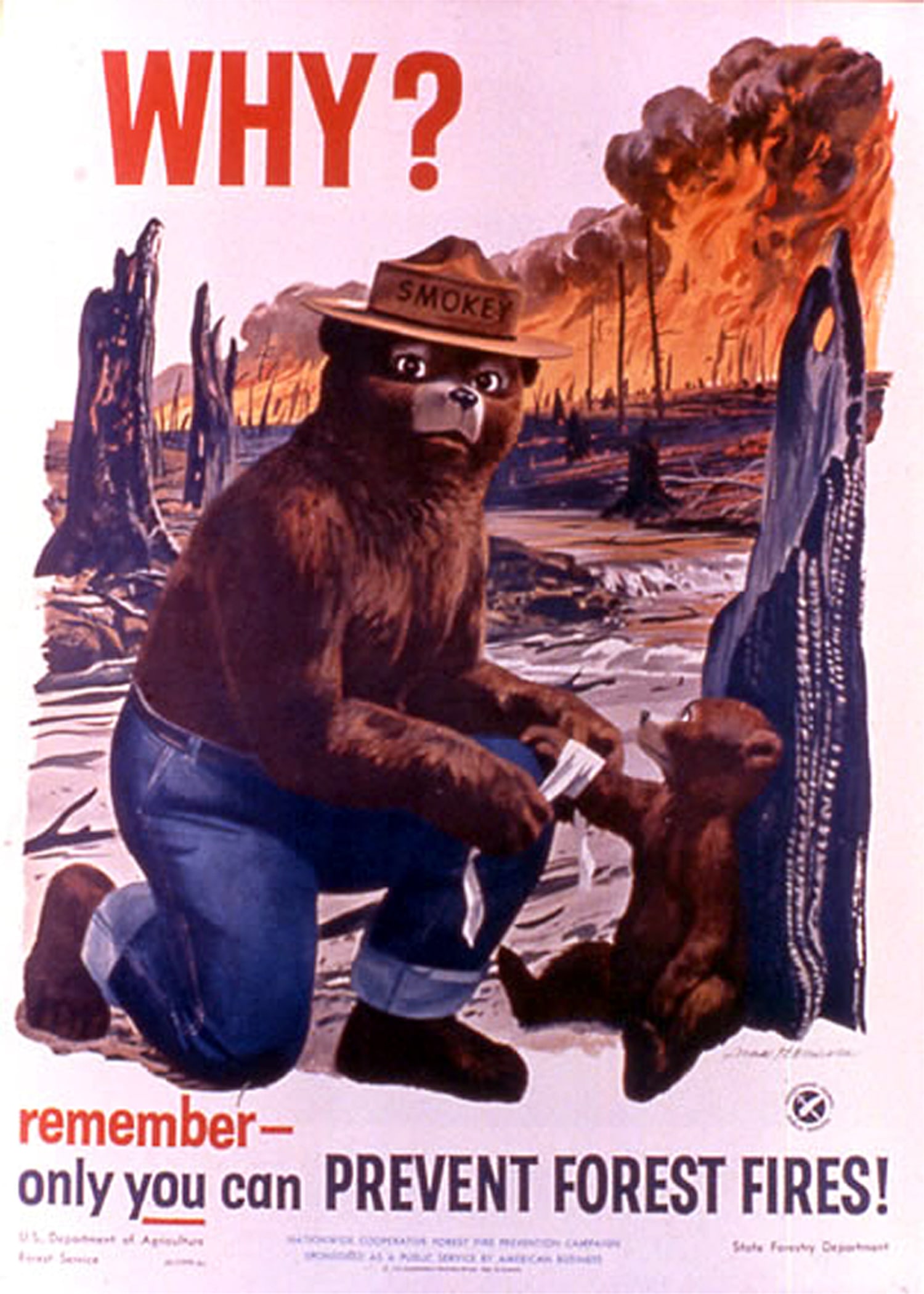This rectangular poster, about five inches high and three to four inches wide, features an illustrated scene vividly capturing the aftermath of a forest fire. Set against a pinkish sky with a raging wildfire in the background emitting orange flames and black smoke, the foreground depicts a poignant moment with Smokey the Bear. Smokey, a recognizable brown bear figure donning a Mountie-style hat labeled "Smokey," blue jeans, and boots, kneels down towards an injured baby bear leaning against a charred tree. With a look of disappointment on his face, he carefully wraps a white bandage around the baby bear's raised right arm, while the little cub gazes back, seemingly thankful. 

The scorched scenery of burnt and broken trees emphasizes the poster's urgent message. Bold red letters at the top left corner ask "Why?", and below in red it states, "Remember," while in black it follows with "Only you can prevent forest fires," with "you" notably underlined in red. The poster also contains fine print at the bottom, which is difficult to read. This striking image and text combination reminds viewers of the critical role they play in preventing forest fires.